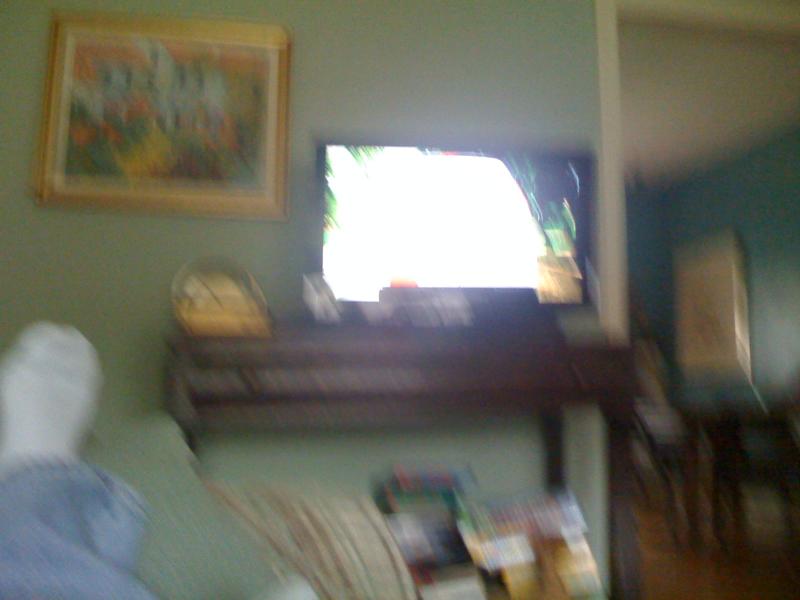The photograph, taken in color and landscape orientation, captures a blurred interior of a cozy living room. In the foreground, to the bottom left, a person reclines on a mint green couch, their leg extending towards the armrest. They are dressed in denim blue jeans and a white sock. The focal point of their gaze is a flat-screen TV, positioned on a dark wooden stand, emitting a bright, indistinct white light that dominates the screen. Above the TV, slightly to the left, hangs a painting characterized by vibrant golds and oranges, adding a splash of warmth to the room. The TV stand also holds a collection of magazines and packages, contributing to a lived-in feel. Beyond this primary space, there is a glimpse of a dining area furnished with a table and chairs, enhancing the depth and homely atmosphere of the scene. The entire image is slightly blurred, suggesting it was captured in motion, adding a dynamic, casual quality to the detailed snapshot of domestic life.